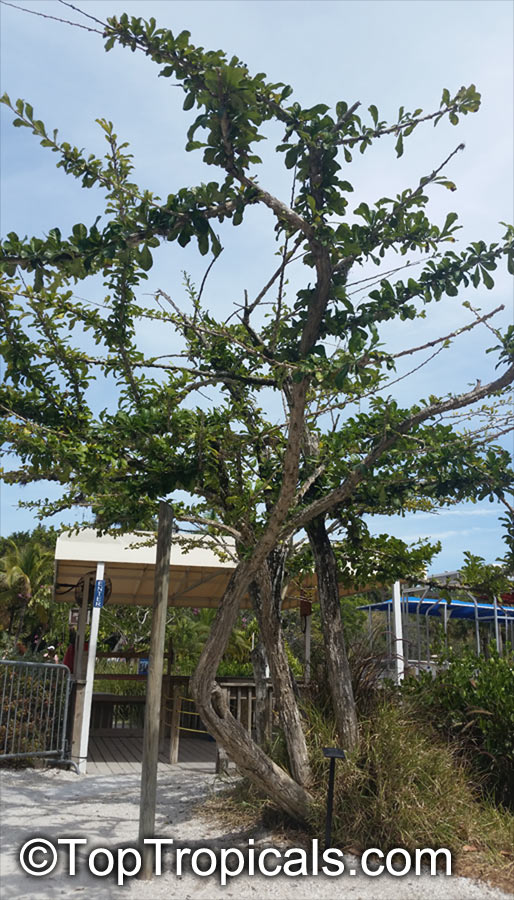This vertical rectangular outdoor scene depicts a unique, multi-trunked tree with an intriguing bend and spread, positioned centrally. Behind it, a pergola-like area with a rope path winds through a wooden setup reminiscent of a bus stop top, though it is not one. To the right, there's a roofed deck area supported by white pillars, with a thin metal roof. Below this roof is a railing and another enclosure in the distance, surrounded by lush vegetation. The foreground features a small metal fence, pavement, and a partially visible post, possibly a light pole. The sky above is bright blue with scattered white clouds. The tree itself stands out with its arching, not fully leafed branches, covered closely by small leaves, and several trunks—one notably curving left before extending upwards. A bush and grass, somewhat unkempt, accompany the scene to the right along a pathway. Notable text at the bottom of the image in white, with a shadow effect, reads "copyright toptropicals.com."